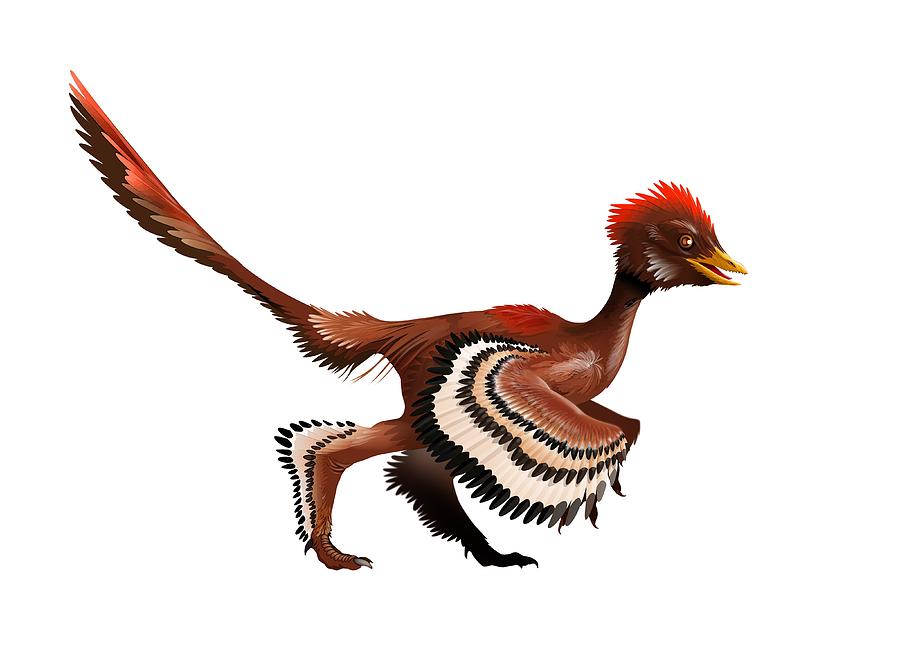The image showcases an animated depiction of a fictional or possibly prehistoric bird-like creature set against a plain white background, prominently centered. This unique animal appears to be reminiscent of a dinosaur-era bird or mini-raptor. The creature is characterized by its vibrant and varied reddish tone, with an overall dark red hue accented by lighter and darker shades. It has a distinctive long tail that points upward at a 45-degree angle, with the tail's tip being light red and the underside a darker brown.

The creature is oriented side-on, facing to the right. It possesses an orange-yellow beak and a striking red mohawk running across its head, complemented by white feathers beneath its eye for contrast. Its legs are bent backward at the knee, resembling chicken feet with sharp claws, feathered halfway down to the claws. The front leg displays white plumage tipped with black, while the back leg features dark black feathers, possibly shadowed.

The wings are intricate and display a spiral-esque arrangement of feathers transitioning from dark brown to black, beige, black again, white, and finishing with black tips. This dynamic creature blends elements of a roadrunner and a feathered dinosaur, though it is an imagined species not found in nature today.